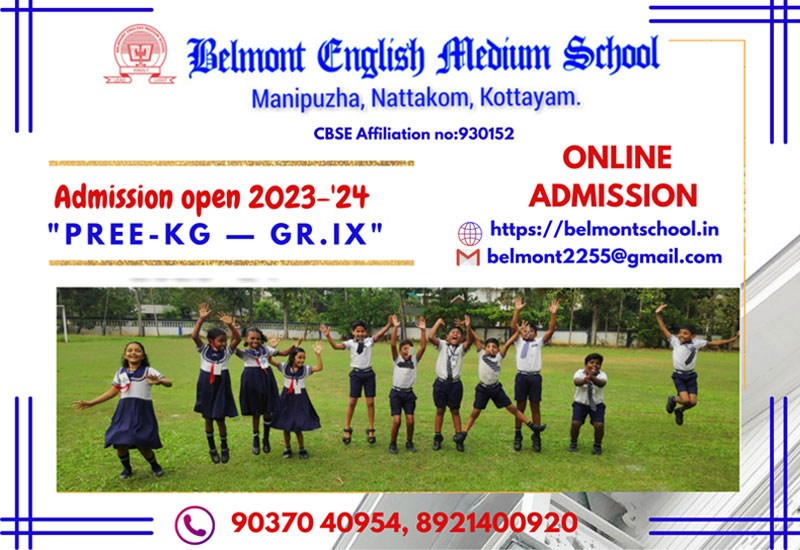This landscape-oriented image features a predominantly white background with a well-organized structure. At the very top, prominently displayed in blue text, is the name "Belmont English Medium School." Below this, the text "Manapusa Natakam Kodayam" is written, followed by the CBSE affiliation number "930152." To the left of this affiliation number, there is a red icon signifying accreditation.

Adjacent to the word "school" is a yellow line that extends horizontally to the right and then descends vertically down the right side of the image, creating a border element. Each of the four corners (upper left-hand, upper right-hand, lower left-hand, and lower right-hand) is decorated with blue parallel lines adding a decorative touch to the edge of the photograph.

Centrally placed within the image is an announcement text: "Admission Open 2023 to 24 PREE-KG-GR.IX." Below this, in red text, is the call for online admission featuring the URL "HTTPS://BelmontSchool.IN" and the email "Belmont2255@gmail.com."

Toward the bottom of the image, there is a vibrant photograph of eleven joyful children with darker skin tones. The children are dressed in charming white uniforms paired with blue skirts and blue shorts, appearing to be having a delightful time.

Lastly, at the very bottom, contact details are provided, marked with a cellphone icon: "9037040954, 8921400920."